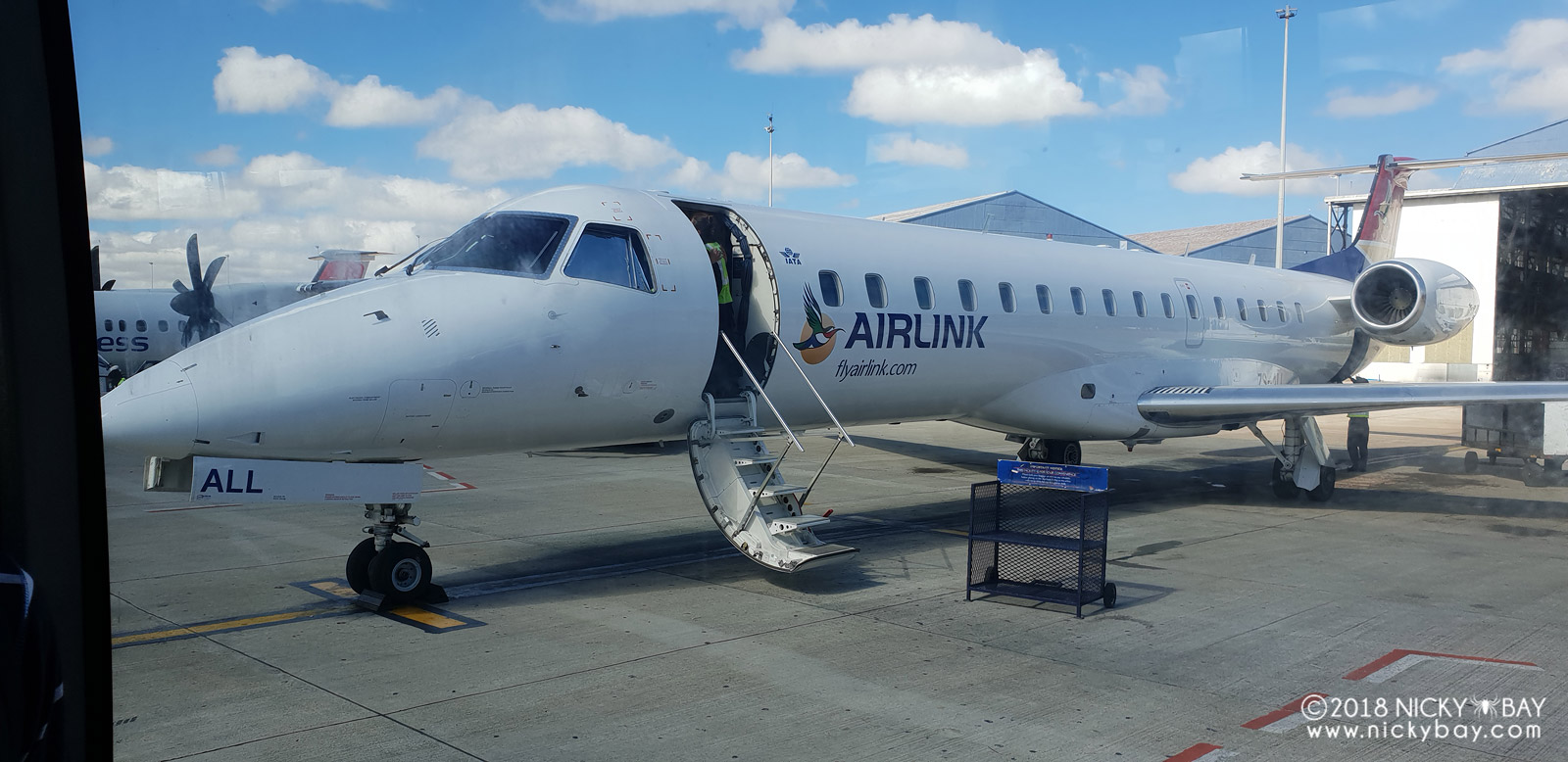The image features a small, white jet prominently displaying "Air Link" and "flylink.com" on its side, adorned with a blue bird on a yellow background. The jet, which can accommodate around 40 people, has a front entrance with a staircase lowered to the gray tarmac, indicating it may be preparing for boarding. The plane's sleek, pointed nose and engine on the left-hand side are clearly visible. Situated at a small airport, the scene includes a nearby hangar, a distant turboprop plane, and a bright blue sky with scattered white clouds. To the right of the jet's stairs is a black metal rolling cabinet, likely for flight attendants' use. Notably, the photograph is credited to 2018 Nicky Bay, as indicated by the logo and website at the bottom of the image.